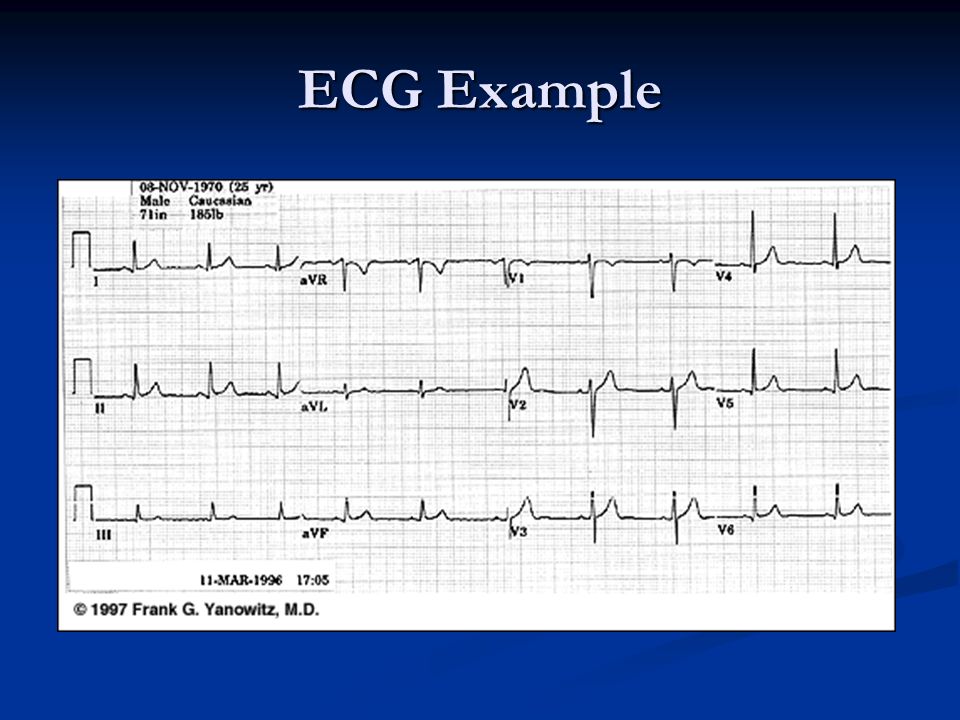The image features a PowerPoint slide with a gradient blue background that fades from dark blue at the top to lighter blue toward the bottom. The title "ECG Example" is prominently displayed at the top in white text. Central to the slide is a white grid displaying three ECG (electrocardiogram) lines that graph the heartbeats. Key details include the documentation of the test: at the top left of the grid, it notes "Male, Caucasian, 71 inches, 185 pounds" with a date of "6 November 1970" and an age of "25 years." Further annotations on the grid mark various points with labels such as "AVR," "V1," and "AVL" along the lines. The bottom left of the grid records the details "11th of March, 1996," at "1705" and "1997 Frank G. Janowitz, MD." The ECG graph lines oscillate distinctly, illustrating the heart’s electrical activity across three rows.